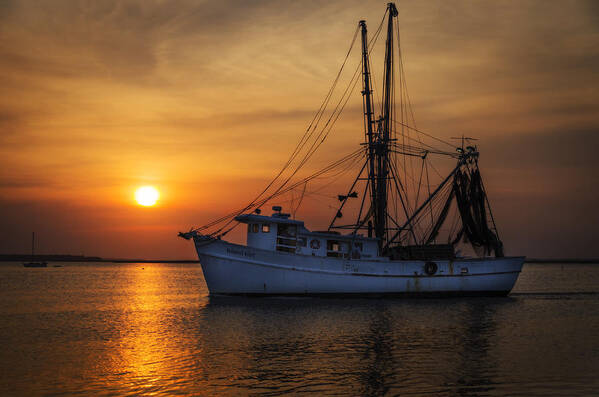This landscape-oriented, color photograph vividly captures a serene evening on the sea, showcasing a weathered, white-painted shrimp boat navigating towards the left. The boat, positioned slightly to the right of center, features two tall masts with extensive rigging and netting angled towards the stern, akin to a classic fishing trawler reminiscent of the one from "Forrest Gump." The boat's surface shows signs of age and rust, adding to its vintage charm. Surrounding the boat, the calm water showcases small ripples and takes on a darker hue, contrasting with the yellowish reflection created by the setting sun. The sun, a bright orange-yellow sphere positioned near the edge of the horizon on the left, bathes the scene in warm tones, while wispy, dark clouds gather around, hinting at the fading daylight. This photograph epitomizes photographic representational realism, offering a detailed and atmospheric snapshot of a tranquil sea voyage at dusk.